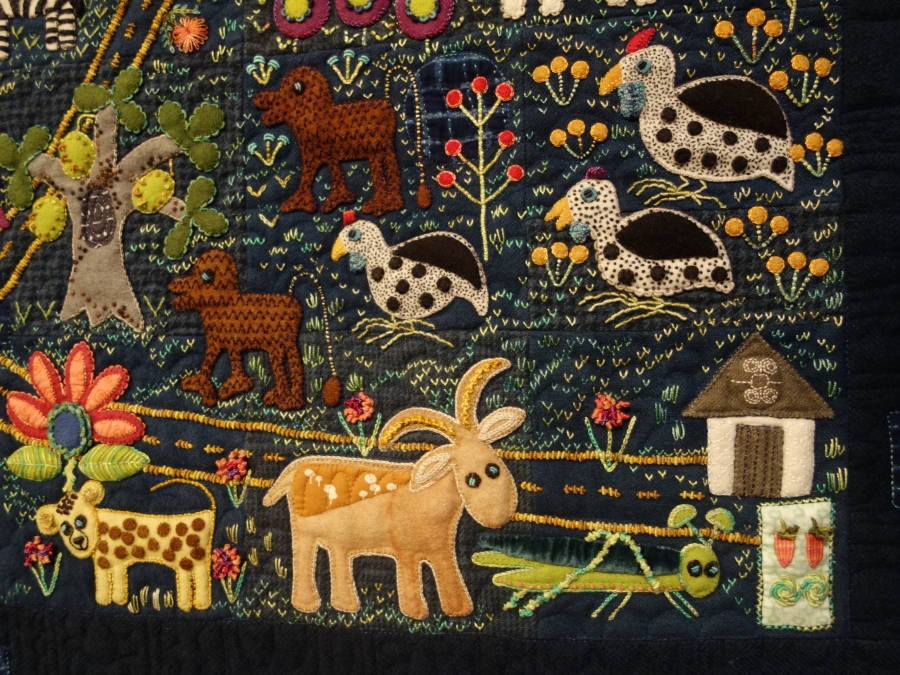The detailed image shows a richly embroidered quilt or tapestry featuring a diverse array of animals, plants, and a small building. Situated at the bottom center is a billy goat or ram, distinguished by its prominent horns and two ears. Adjacent to the goat on the right is a meticulously stitched grasshopper, while to the left stands a uniquely depicted giraffe with a notably short neck, possibly mistaken for a lion or leopard by some observers. The scene includes three intricately designed chickens, each with scales and polka dots, small red crests, yellow beaks, blue necks, and little giblets under their necks, positioned in the upper right section. These birds have black wings or backs adorned with white dots. To the left of this group, two brown animals with distinct features—possibly dogs with blue eyes, large feet, big mouths, and long, puffy tails—are visible. In the background, a small shed or building with a path leading from it adds depth to the composition. The left side of the image features a tree bearing what appears to be three different types of fruit, while a monkey is positioned near it. The tapestry's dark green to black background is accented with plants and flowers, and in the top left corner, part of a zebra's tail and legs can be seen. The overall composition, mostly in hues of blue, is a testament to artistic creativity and attention to detail.